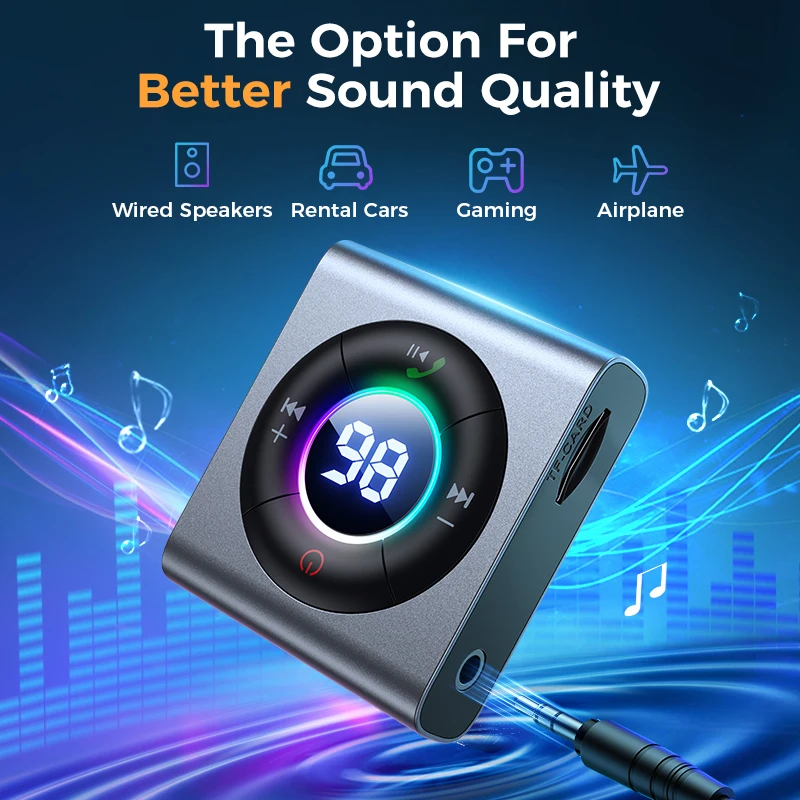**Unleash Superior Sound Quality with the Ultimate Audio Companion**

Experience unparalleled audio quality with our latest device, reminiscent of the iconic iPod Nano. Set against a sleek blue backdrop adorned with vibrant musical notes and audio waveforms, this compact square gadget is showcased in a crisp, clear photograph that exudes modern sophistication. 

Prominently featuring the tagline "The best option for better sound quality," this versatile device caters to all your audio needs. It is equipped with a dial at the center that not only adjusts volume but also allows you to navigate through your music or recordings effortlessly. Notably, the dial features a phone handle icon, hinting at its capacity to sync with your phone for seamless call management.

Designed with practicality in mind, this device includes an auxiliary jack that connects to wired speakers for an immersive home audio experience. In addition, it's perfect for on-the-go listening, easily plugging into your car’s audio system to replace mundane radio with your personalized playlists. It also mentions "rental cars," highlighting its portability for travelers. 

Gamers and frequent flyers will find solace in the mention of "gaming" and "airplane," indicating versatility and convenience. Whether you're indulging in some in-flight entertainment or immersing yourself in a gaming session, this device ensures high-fidelity sound.

For a touch of elegance, the text "better" is highlighted in orange, drawing attention amid the otherwise white typography. The number 98 appears on the device's interface, adding to its modern aesthetic.

This promotional page presents an all-in-one solution for superior sound quality, demonstrating that good things do come in small, impeccably designed packages. Make every moment sound better with this essential audio accessory.